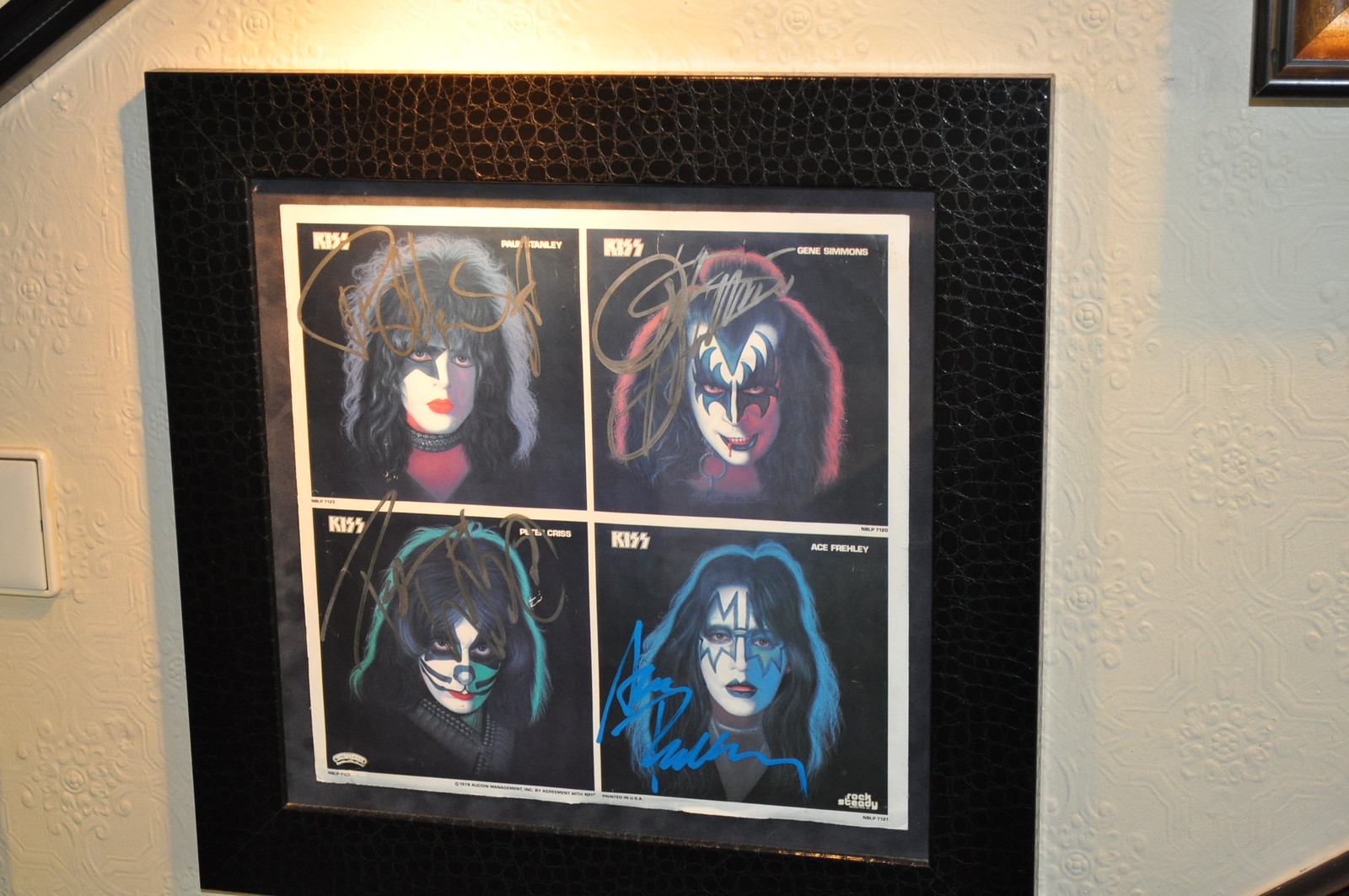The image features a detailed close-up of a framed collage depicting illustrated headshots of the four members of the band KISS. The frame itself is made of black leather with a scaly, snakeskin-like texture, set against a white wall with a decorative texture and illuminated by overhead lighting. In the collage, each quadrant showcases one band member, identifiable by their iconic makeup and hairstyles. The upper left portrait features a member with black hair, a star painted over one eye, white face paint, red lips, and a collar, accompanied by a possible autograph. To the right, another member with a mohawk and long sides, sporting dark blue makeup around the eyes that forms spikes, black lipstick, and a menacing downward gaze, also bears an autograph. In the lower left, a member with black hair and bangs has diamond-shaped black eye paint, black paint around the nose resembling whiskers, and another autograph. The lower right image shows a member with black outlined spikes over the eyes and black painted lips, similarly autographed. Each image has a white border and a black internal border that complements the textured black frame. The framed collage is part of a larger arrangement, with additional frames partially visible around the main image.